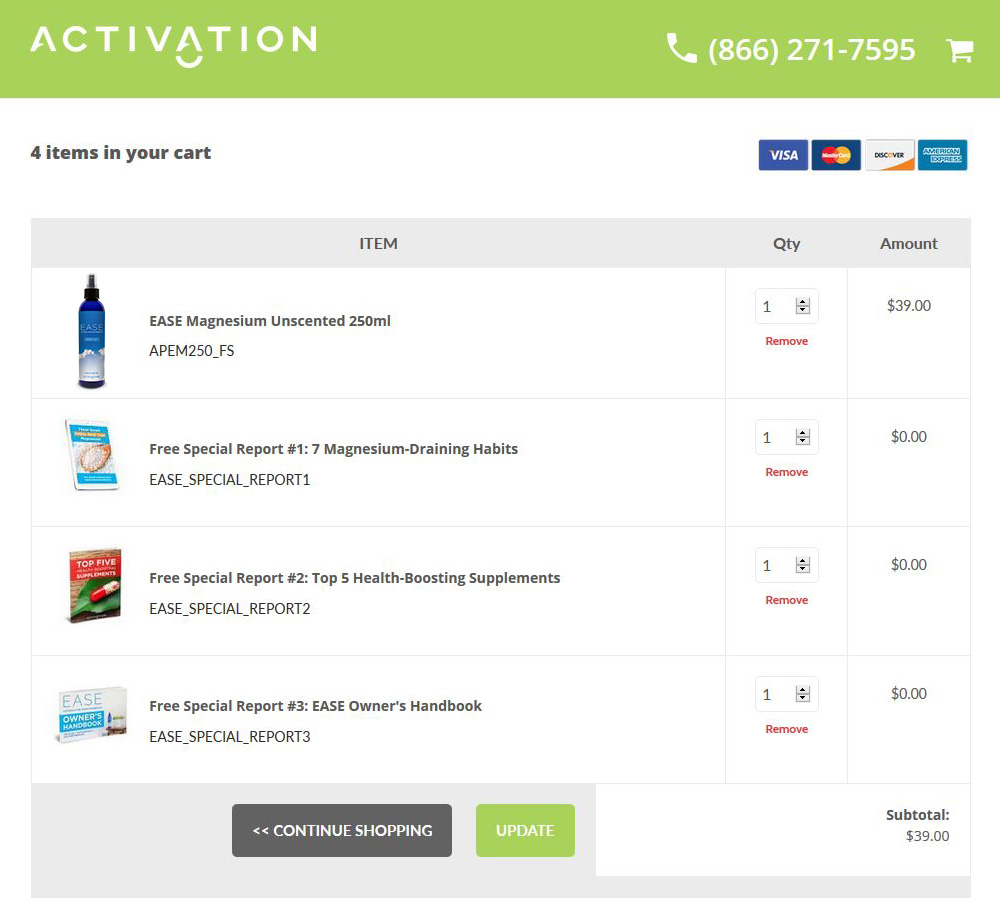The image depicts the storefront webpage for a store called "Activation," featuring a prominently displayed phone number (866-271-7595) at the top of the page. This contact detail is flanked on the right by a shopping cart icon and on the left by a phone icon. These elements are all set against a green rectangular banner. The shopping cart indicates that there are four items currently in the user's cart.

On the right side of the page, four payment logos—Visa, MasterCard, Discover, and American Express—are neatly arranged. 

The cart contents are detailed as follows:
1. Ease Magnesium Unscented (250 milliliters) priced at $39, with a quantity of one.
2. Free Special Report #1: "Seven Magnesium Training Habits," priced at $0 with a quantity of one.
3. Free Special Report #2: "Top Five Health-Boosting Supplements," priced at $0 with a quantity of one.
4. Free Special Report #3: "Ease Owner's Handbook," priced at $0 with a quantity of one.

The subtotal for the items is listed as $39. Below the items, there are two clickable buttons: "Continue Shopping" and "Update."

Each item listed in the cart is accompanied by a relevant image: a blue bottle for the Ease Magnesium Unscented, a blue e-book cover for the first special report, a red and green e-book cover for the second special report, and a white and blue e-book cover for the third special report.